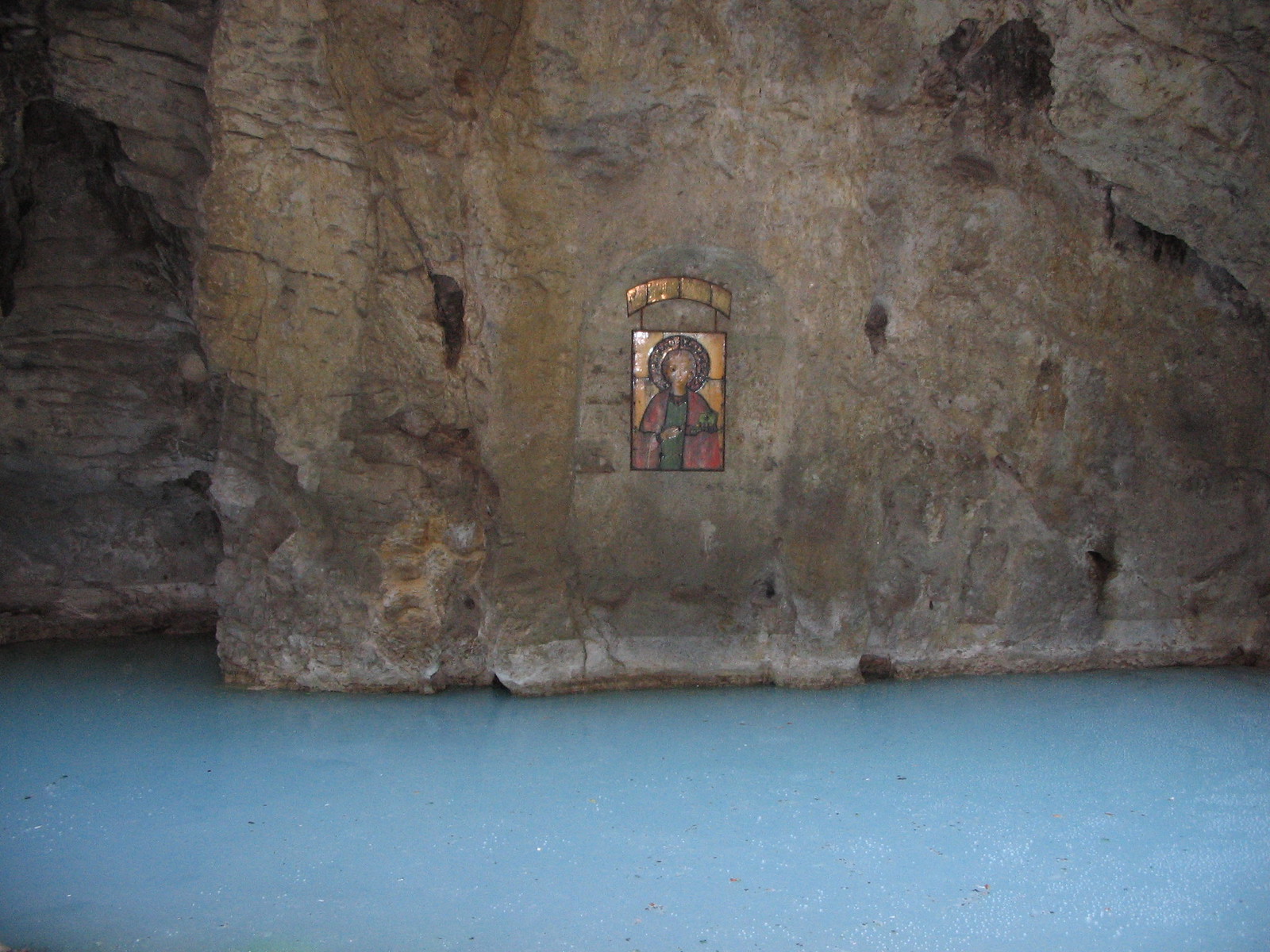This rectangular photograph appears to have been taken inside a cave or potentially a man-made cavern. The cave’s jagged yet flat rock walls exhibit a mix of grays, browns, and subtle orange and white tones, giving a rugged and textured appearance. In the center of the cave's rear wall, there is a notable art piece, which might be a painting or a stained glass window. This artwork seems to feature a woman, possibly the Mother Mary, adorned with a halo and wearing distinctive attire. The lower section of the photograph showcases a smooth, light blue surface, which could either be very still water or a shiny concrete floor. Adding to the ambiance, a gold arch frames the artwork, enhancing its religious and ornate character. The entire scene melds natural elements with man-made modifications, creating a visually intriguing and serene atmosphere.